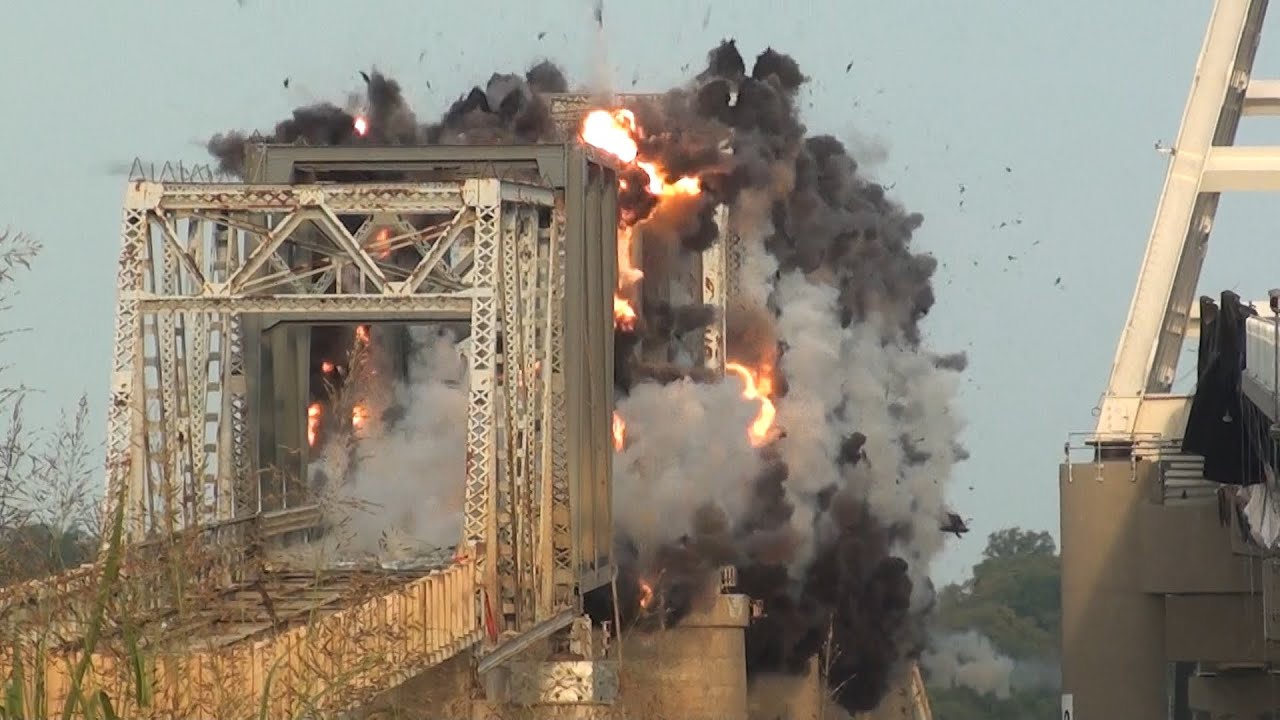This is a horizontal, rectangular image capturing the dramatic scene of a metal bridge engulfed in flames and smoke. The front opening of the bridge is visible, but beyond that, the interior is obscured by a chaotic mix of bright orange and yellow flames, thick black smoke concentrated at the top, and billowing white and gray smoke. The bridge, with its metal structure and golden hue, stands taller than the trees visible in the lower background, which are set against a gray sky. To the side of the bridge is another structure featuring a concrete base and metal girders extending upwards. The scene suggests a possible planned demolition, with debris and explosive energy filling the air, including intense columns of smoke rising up. The image's clarity of the day highlights the stark contrast between the bridge's fiery destruction and the otherwise calm surroundings.